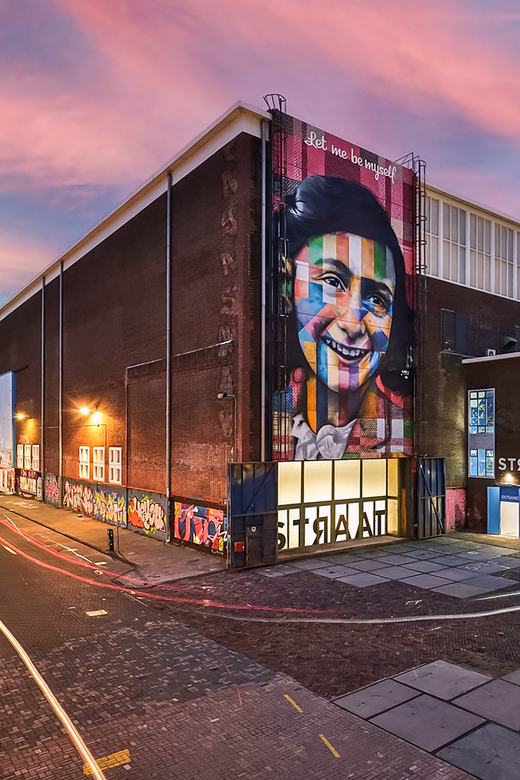In this outdoor photograph, the focus is on a somewhat dilapidated red brick building with various forms of artwork and text. In the foreground, square concrete tiles create a walkway leading up to the building. The centerpiece of the building is a large, vibrant mural of a young woman’s face painted in striped colors of red, green, blue, white, yellow, and purple. Above the mural, the white text "Let Me Be Myself" is prominently displayed. To the left side of the mural, the building has graffiti at the bottom, adding to its weathered look. The windows in the building are illuminated, suggesting the time could be around sunset, as evidenced by the purple and pink hues in the sky. The structure also features the word "STR AAT" in what appears to be either Russian, Dutch, or German text, hinting that this building is likely located outside of the United States. Despite its neglected appearance, the mural adds a significant artistic touch, possibly a depiction of Anne Frank, contrasting with the urban decay of its surroundings.